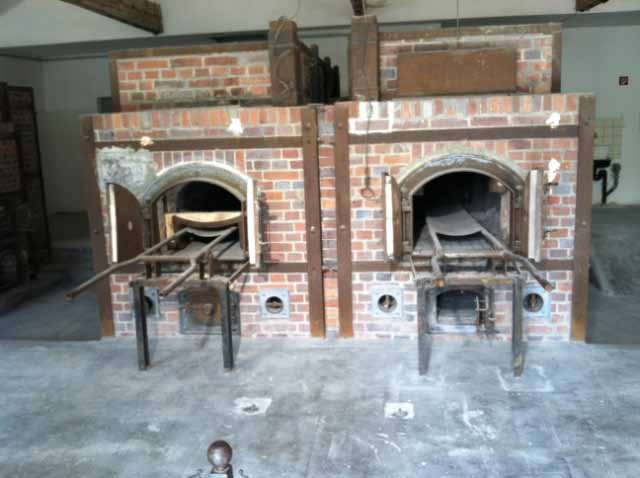This is a detailed photograph featuring two side-by-side, old-fashioned brick ovens that dominate the center of the image. Both ovens, constructed from red and gray bricks, extend from the floor to the ceiling of the room, evoking a utilitarian, industrial ambiance. The backdrop is a stark, plain white wall that contrasts with the gray slate floor. Each oven has open doors, and inserted into these are long, metal trays with handles—tools that seem designed for sliding items in and out of the ovens.

Below the oven doors are square openings that suggest these could be areas for placing fuel, possibly coal. To the left side of the image, there's a darkened area that appears to be a doorway. Additionally, a metal or brass railing post is visible at the bottom of the photo, hinting at a barrier likely meant to keep viewers at a distance, emphasizing the historical or significant nature of the ovens. This photograph captures an antiquated design, with implications that it could be a modern-day crematorium or a historical site, possibly eliciting strong associations with grim historical uses.